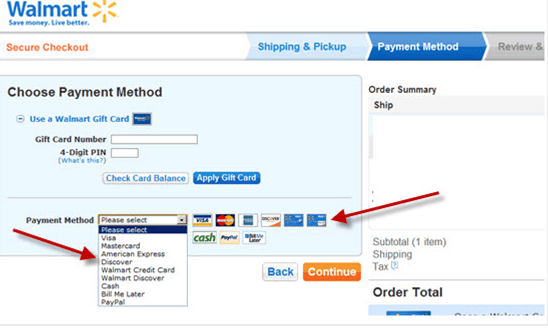The image depicts an outdated version of Walmart's online checkout process. The background is white, and in the top-left corner, the Walmart logo is displayed in blue text with the tagline "Save Money. Live Better" also in blue. To the right of this text is the Walmart star-shaped symbol in a golden-yellow color. Below this, there's a gray bar with a white center, labeled "Secure Checkout" in orange text. 

This gray bar includes a navigation trail for the checkout steps: Shipping and Pickup, Payment Method, Review, and an obscured fifth step on the far right. In the center-left portion of the image, there's a light blue box titled "Choose Payment Method." This box provides options to use a Walmart gift card, with fields to enter the gift card number and PIN, check the card balance, or apply the gift card.

Underneath the gift card section, there's a "Payment Method" dropdown box, with 'Discover' indicated, highlighted by a red arrow. In the right section of this dropdown, an image of a Discover card is pointed out by another arrow. On the right side of the image, there's an order summary and total section, while at the bottom center of the image, there's a "Back" button to return to the previous step and a "Continue" button to proceed with the checkout.